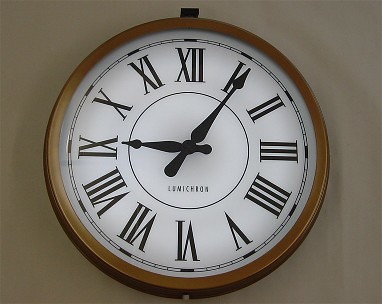The image depicts a traditional, circular clock with a white face and black hands. The clock prominently features black Roman numerals indicating the hours, with small black markings around the periphery to accentuate each hour further. Encircling the face is a distinctive black and white pattern that adds an elegant border. At the center of the clock, a fine black line is seen, likely a design element, and beneath the clock hands is some writing, presumably indicating the manufacturer's name.

The clock is framed in an elegant gold-brown color, giving it a distinguished look. It is suspended from the top by a small black hanging device. There is a screw visible at the lower edge of the clock, which is likely used to remove the face for battery replacement or maintenance. The clock is mounted on a light brown wall, and there are no other objects or elements visible in the image, centering the viewer's attention entirely on the clock.